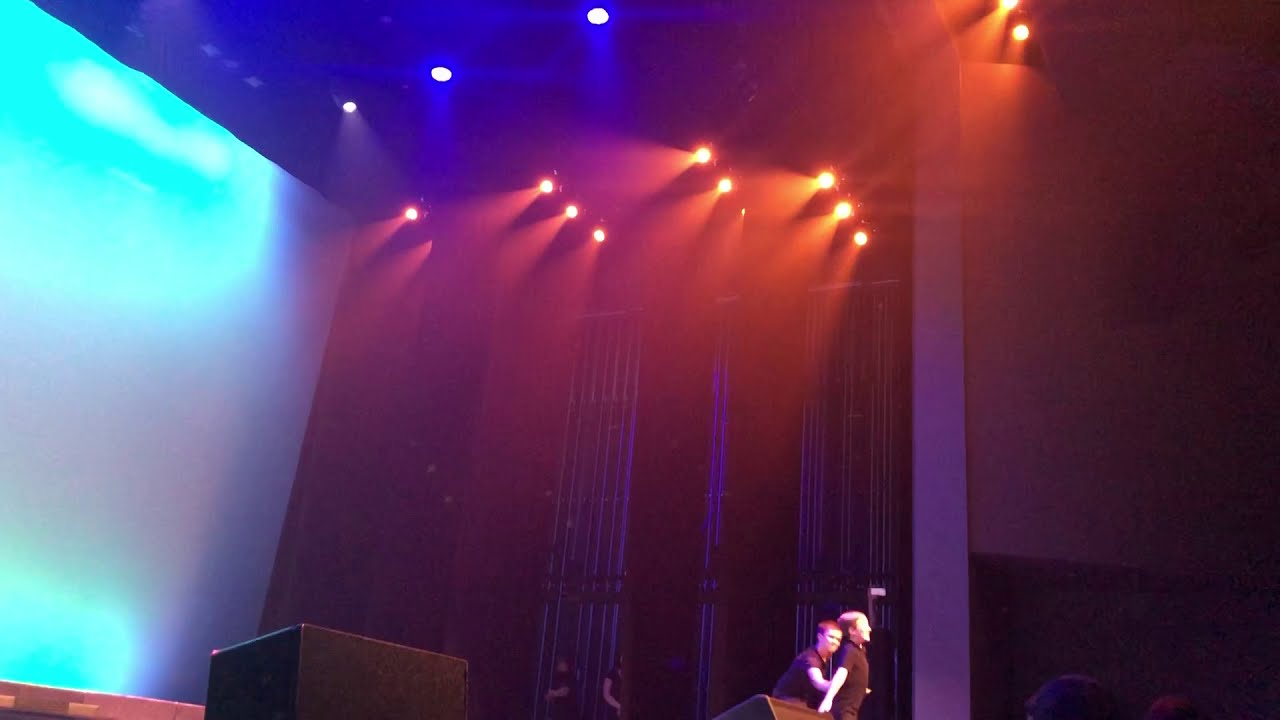In the photograph, set inside a dimly lit theater, two young white individuals, possibly children, stand on stage dressed in black outfits. The stage backdrop features a large blue screen illuminated by a set of five spotlights. Bright yellow and blue lights shine from above, mounted alongside red and blue lights in the rafters, and a pair of big black speakers flank the stage. The ceiling and walls of the theater are predominantly black, with some pipes and walls in silver and gray tones. One of the children, with fair hair, looks directly at the audience with arms spread wide, while the other, possibly a boy with brown hair, hugs him from behind, clasping his waist. Additional monitors and floodlights are positioned at the front of the stage. In the background, two other individuals dressed in black can be faintly seen, as well as a sparse seated audience. The setting is clearly an indoor venue designed for onstage performances.